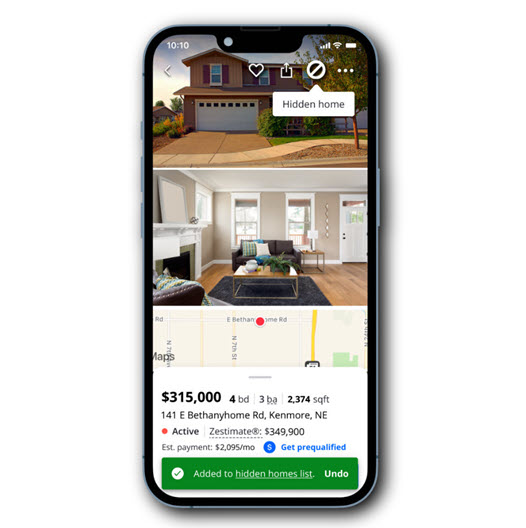In this image, a smartphone is displayed face-up showing a real estate application screen. At the top of the screen, the time is displayed as 10:10. The main feature of the display is a computer-generated image of a two-story home with a white garage. Accompanying the image are three icons in the upper right corner: a heart, a download arrow, and a circle with a diagonal slash through it. 

Below the home image, the text "Hidden Home" is prominently displayed, followed by a photograph showing the interior of a living room. The living room features a white-mantled fireplace, a dark gray rug centrally located, and a wooden and metal coffee table. In the background, a dark gray loveseat adorned with throw pillows is visible.

Further down, there is a map with a red circle indicating a specific location near the top center. Relevant property details are listed below this map, including the price of $315,000, specifications of four bedrooms, three bathrooms, and a total of 2,374 square feet of living space. The address provided is 141E Bethany Home Road, Kenmore, NE. Additional information includes the status of the property as "Active," a Zestimate of $349,900, an estimated monthly payment of $2,095, and a "Get Pre-Qualified" prompt.

At the very bottom of the screen is a green rectangular button, featuring a white circle with a green checkmark inside it, and the text "Added to Hidden Homes List, Undo."